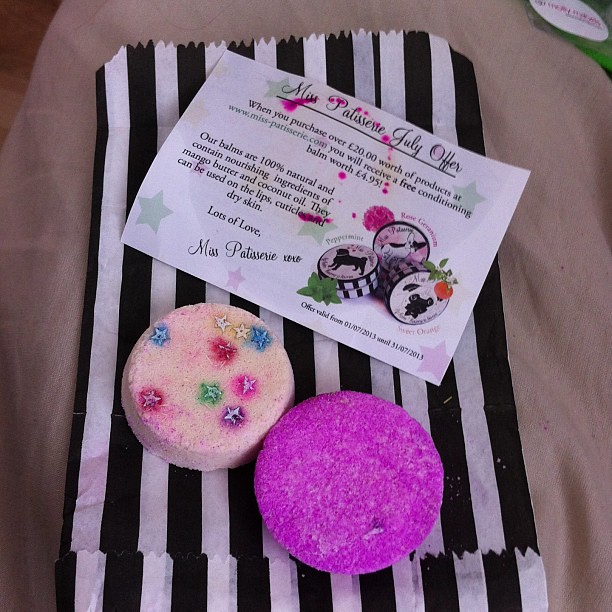The photograph displays an arrangement of bath and skincare products artistically set on a camel-colored blanket. Central to the image is a black and white vertically striped paper bag. Positioned across the bag are two bath bombs, one being a deep lavender purple and the other beige adorned with colorful stars. Lying diagonally above the bath bombs is a rectangular white piece of paper featuring details about a Miss Patisserie promotional offer. The text reads: "Miss Patisserie July Offer: When you purchase over £20 worth of products at www.miss-patisserie.com, you will receive a free conditioning balm worth £4.95. Our balms are 100% natural, containing nourishing ingredients such as mango butter and coconut oil, suitable for lips, cuticles, and dry skin. Lots of love, Miss Patisserie, XOXO." Additional information includes product descriptions like body butters in Peppermint, Rose Geranium, and Sweet Orange, with the offer valid from 01-07-2013 to 31-07-2013. The serene setting and the detailed description evoke a sense of luxury and relaxation, emphasizing the natural and artisanal quality of the products.